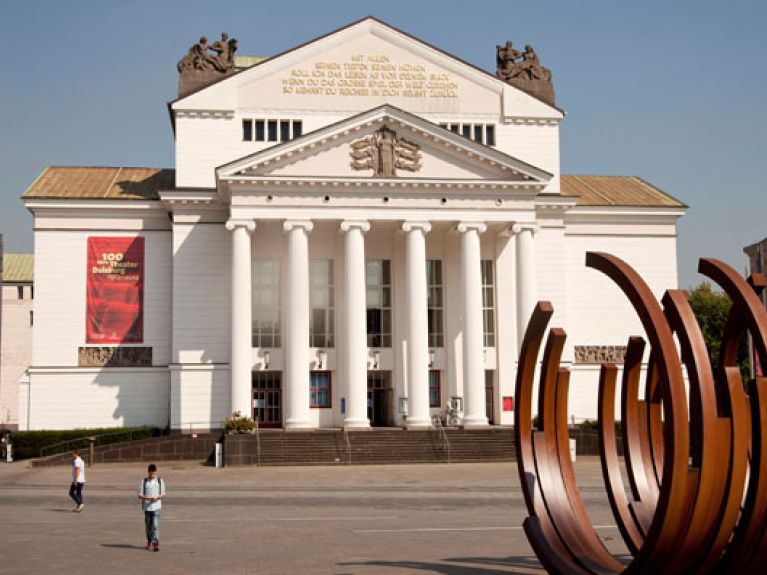The image depicts the exterior of a grand white brick theater building on a clear blue day. This three-story structure features a prominent portico supported by six large white columns, with a red banner indicating it is a theater, displaying partially visible text that suggests "theater" and "100". At the top of the building, the gable includes some unreadable writing. Crowning the peaked roof above the portico are two statues situated at the corners. The front facade showcases windows covering the second floor, and doors on the first floor, partially hidden behind the columns.

In front of the building, there is a wide staircase consisting of three rows of concrete steps leading down to a gray parking lot where a few people are visible, some walking towards the camera and others toward the left. Additionally, a wheelchair-accessible ramp extends from the left side of the staircase into the parking lot area. 

Prominently placed in the foreground is a distinctive outdoor sculpture made up of a series of incomplete circles, resembling wooden rings arrayed side by side, contributing to the artistic ambiance of the scene. The image captures a bright, serene day with a clear blue sky, emphasizing the detailed architectural and artistic elements of the theater building and its surroundings.